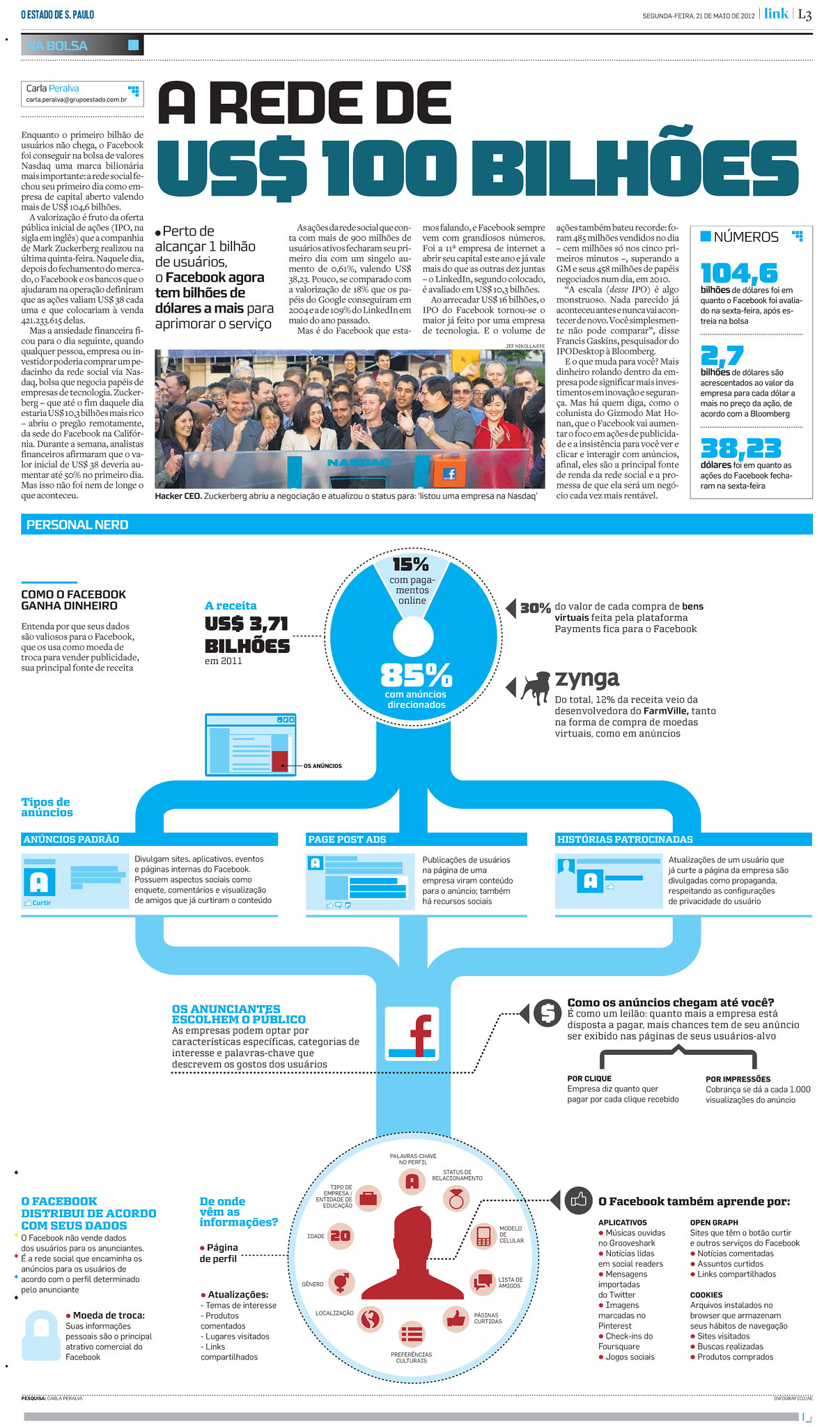This image appears to be a page from a magazine or potentially a web page, indicated by the dimensions and layout described, more vertical than horizontal. On the upper right corner, it is marked "L3" with the word "link" next to it. The content is not in English but seems to be in Spanish. The top part features a headline which mentions "a hundred billion" and an article comprising a few columns of text with blue-highlighted numbers.

Below the article is a photograph showing several people standing behind a large podium, prominently displaying the Facebook logo. The bottom section showcases a large blue diagram: a combination of pie charts, boxes with various charts, and a circle segmented into categories. The diagram includes references to Zynga, Farmville, and again, Facebook, implying it discusses various activities related to Facebook users and their engagement on the platform. The arrangement and the blue-colored visuals underline statistical information, likely representing data points and percentages related to social media usage.